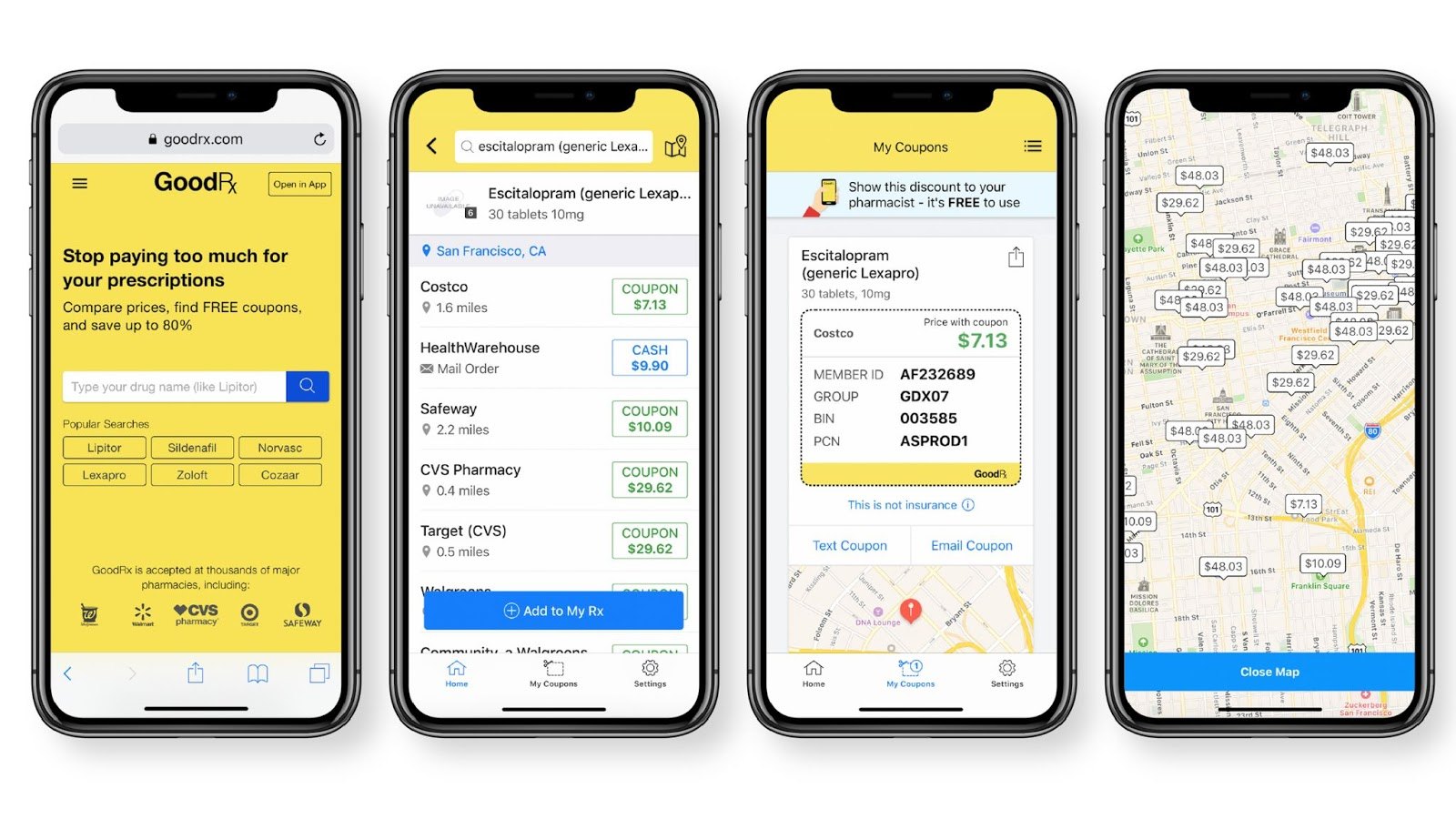The image displays four cell phones, each showcasing a different screen related to prescription cost savings, specifically through the GoodRx platform. 

1. **Leftmost Phone**: This screen features the GoodRx homepage, highlighted with a bold yellow background. The headline reads, "Stop paying too much for your prescriptions." Below this, it encourages users to "Compare prices and free coupons and save up to 80%."

2. **Second Phone**: The upper portion of this screen also has a yellow background. It displays information for "Equispatol PRAM," a generic form of Lexapro. Listed details include a quantity of "30 tablets" at "100 milligrams." Further down, the screen provides a list of pharmacies showing where the medication is available, along with coupon details.

3. **Third Phone**: This screen transitions to the "My Coupons" section. It advises users to "Show this discount to your pharmacist" and emphasizes that the service is "free to use." A coupon is displayed prominently with the text, "Price with coupon: $7.13."

4. **Rightmost Phone**: Featuring a map, this screen shows various locations where the listed medication can be purchased, along with the respective prices at each pharmacy. 

Overall, the four screens collectively illustrate a step-by-step process of searching for, selecting, and utilizing discounts for prescription medications using GoodRx.